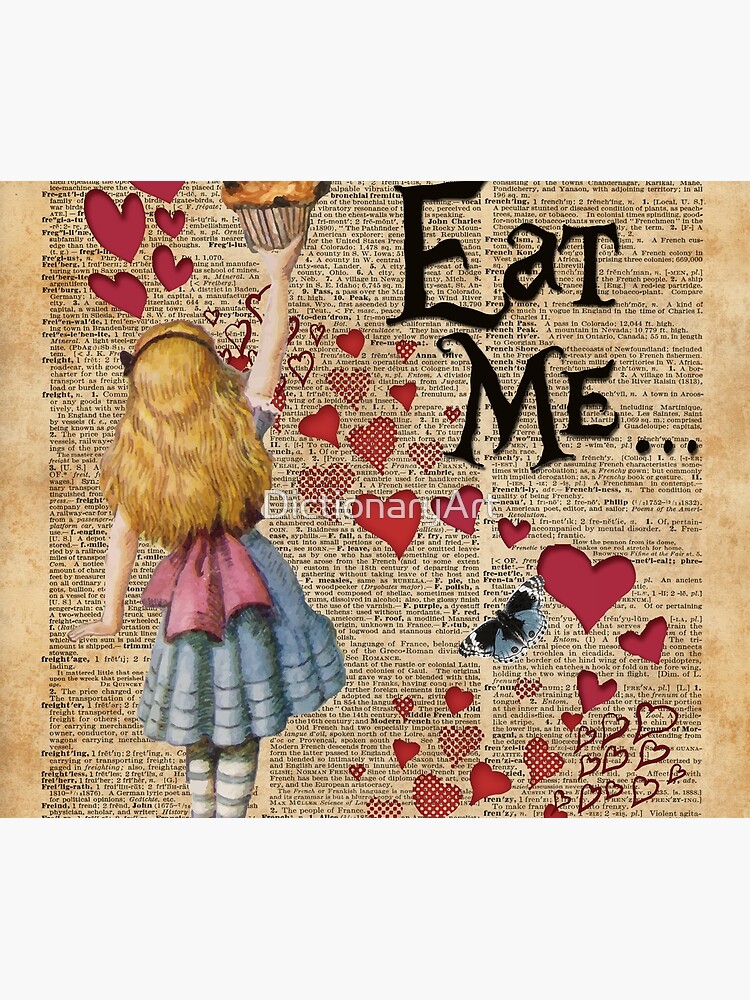This image showcases a unique piece of dictionary art, featuring a dictionary page as the canvas. The dictionary page, filled with black text defining words from the F category, forms the intricate background. Painted on this page is a young girl with her back to the viewer, reminiscent of Goldilocks, wearing a light blue dress with ruffles at the bottom and a large red ribbon around her waist. Her long blonde hair cascades down her back, and she has a headband adorning her hair. Reaching up with her right hand, she grasps a large cupcake, nearly out of the frame, adding a whimsical charm to the scene. She also wears white stockings with blue horizontal stripes.

Adding to the playful nature of the artwork are numerous hearts in red, red and white, or red with white polka dots, which span from the upper left corner down to the lower right of the image. Additionally, a blue butterfly is subtly painted in the bottom right corner. The entire artwork is overlaid with the words "eat me..." printed boldly in black in the upper right corner, inviting a sense of curiosity and fantasy. Clear in the center of the image, the term "dictionary art" emphasizes this artistic form of turning dictionary pages into imaginative scenes, possibly rendered with watercolors or colored pencils.